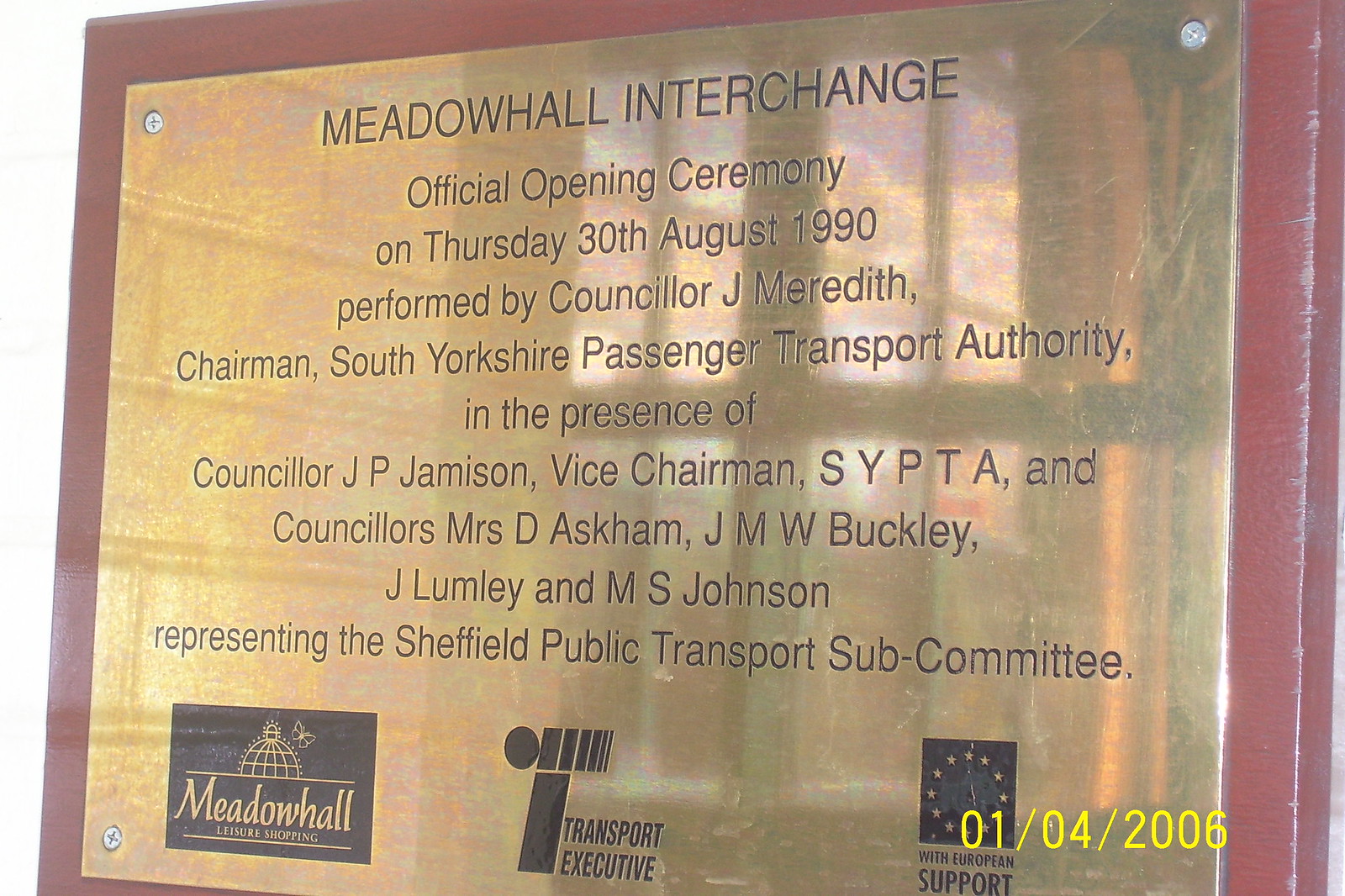The image depicts a reflective, gold metal plaque mounted within a red frame, situated on a maroon-colored wall. The plaque commemorates the official opening ceremony of the Meadowhall Interchange, which took place on Thursday, 30th August 1990. The ceremony was performed by Councillor Jay Meredith, Chairman of the South Yorkshire Passenger Transport Authority, in the presence of Councillor J.P. Jameson, Vice-Chairman of SYPTA, and Councillors Ms. Dee Askham, J.M.W. Buckley, J. Lumley, and M.S. Johnson, who represented the Sheffield Public Transport Subcommittee. The bottom left of the plaque features the Meadowhall Leisure Shopping logo, and in the center bottom is a Transport Executive logo. On the bottom right, there is a logo indicating European support. The photograph’s timestamp in yellow, '1-4-2006,' is visible in the bottom right corner. The plaque also reflects surrounding windows and potentially a building behind the viewer.